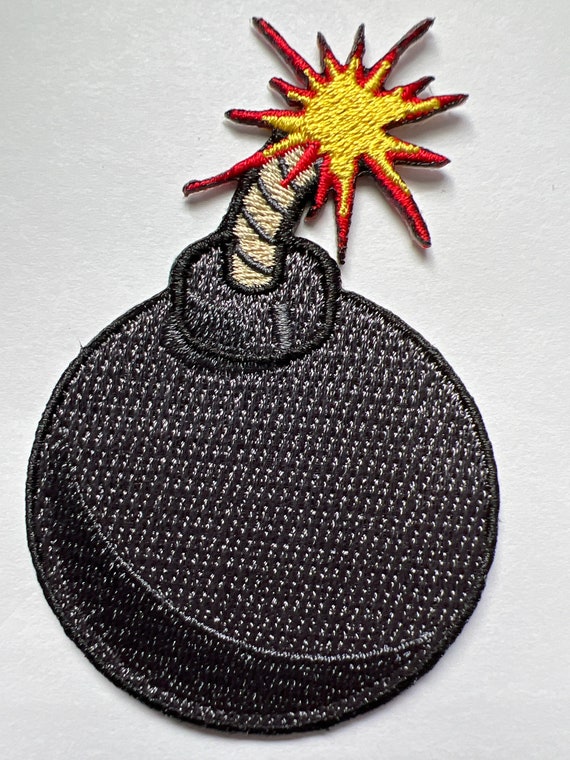The image displays a meticulously hand-sewn embroidered patch lying on a smooth, white background. The patch is designed to resemble a cartoon-style bomb, featuring a large, round black sphere with intricate black stitching for added texture and detail. Above the sphere is a fuse, characterized by light yellow with black stripes running horizontally. This fuse is lit, leading to an explosion depicted at its tip. The explosion is intricately crafted, featuring a starburst-like pattern with about 10 to 15 varying points. The outer edges of the explosion are outlined in red and black, while the inner area glows with a bright yellow. The detail and craftsmanship of the patch are evident, making it a striking visual piece suitable for affixing to clothing or accessories.